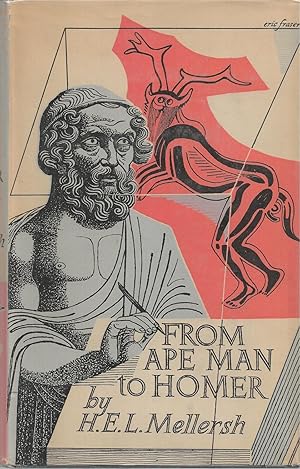The image depicts the cover of a book titled "From Ape Man to Homer" by H.E.L. Mellersh. The cover is predominantly soft pink with coral pink accents. Dominating the left side of the cover is a man resembling a Roman or Grecian statue, with curly hair, a curly beard, and a toga draped over his left shoulder, exposing his pectoral and bicep muscles. He holds a pen in his right hand, which points to a tablet inscribed with the book’s title and author. Behind him, on the right side, is a mythological creature, outlined in black, set against a red backdrop. This creature features a peculiar combination of human and animal traits: antlers, long ears, a bearded or cat-like face, and a monkey-like tail. The name "Eric Fraser" appears in black in the top right corner. The cover is framed with lines that form a square around the artwork.